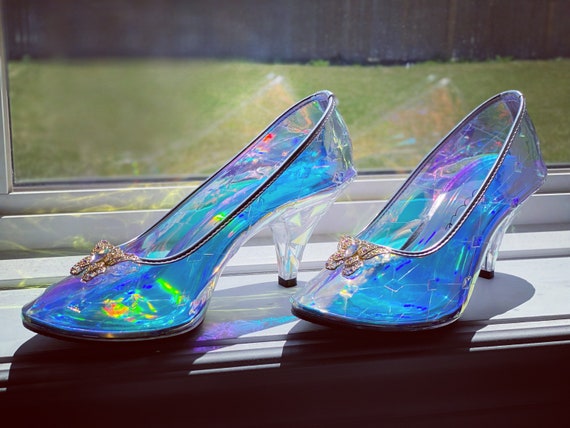In this image, we see a pair of elegant, glass-like blue pumps with clear heels, each adorned with an ornate silver butterfly design at the front. The shoes are positioned on a white wooden windowsill, against a backdrop of a green lawn and a wooden fence, which can be seen through the window behind them. The material of the shoes shimmers with reflections of green, red, orange, and purple, adding to their sparkling, iridescent quality as light passes through them. The intricate silver trim lines the inner part of the shoes, enhancing their ornate appearance. The well-kept backyard outside offers a serene, contrasting background to the glamorous footwear.